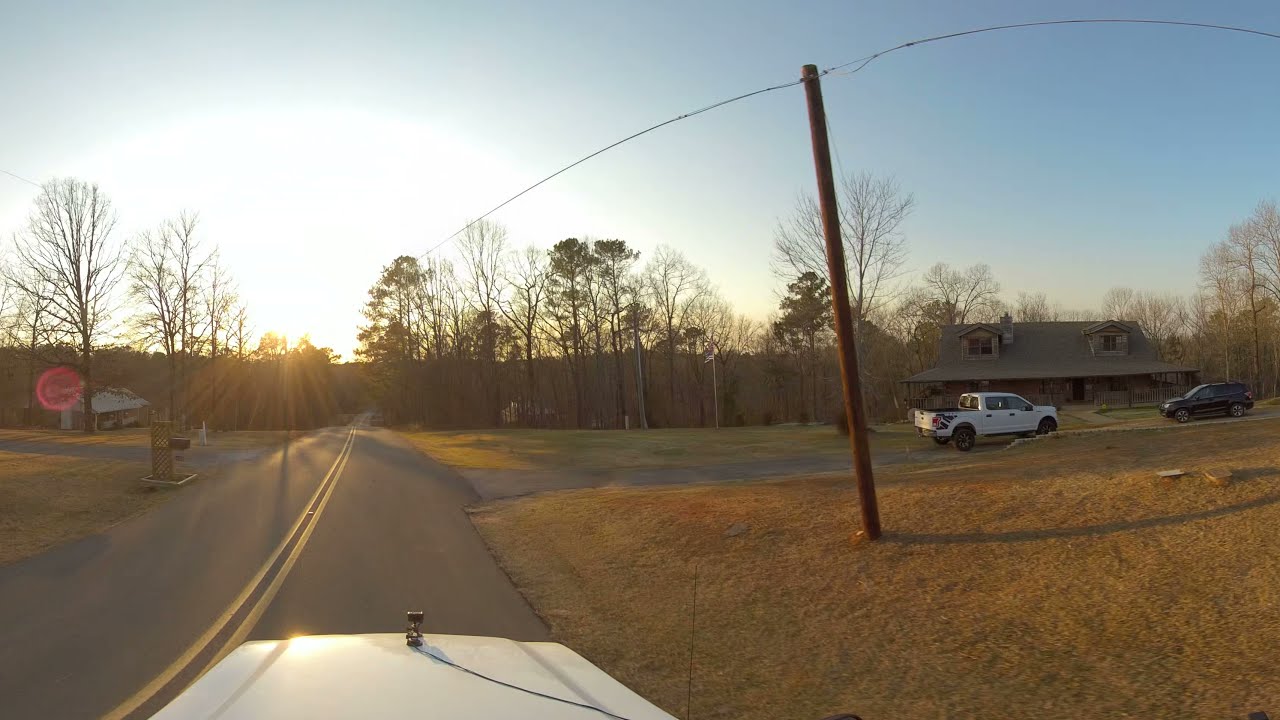The image captures the perspective of someone driving an older-style white car, possibly a Cadillac or Lincoln, down a two-lane, paved road with a yellow divider. The view is through the windshield, and you can see part of the car’s hood with an ornament. It's either evening or approaching dusk, casting a subdued light on the surroundings.

To the right of the road, there is a driveway leading up to a house with a dark brown exterior and second-story windows. Two vehicles are parked near the house: a black car and a white truck that resembles a Suburban. In the background, a mix of trees with varying states of foliage—some lush and green, others bare and dark—clusters around the house, adding depth to the setting. There are electric poles with wiring visible, and in the distance, the sun can be seen low on the left horizon. The scene evokes a small town atmosphere, tranquil yet detailed with lifelike elements.